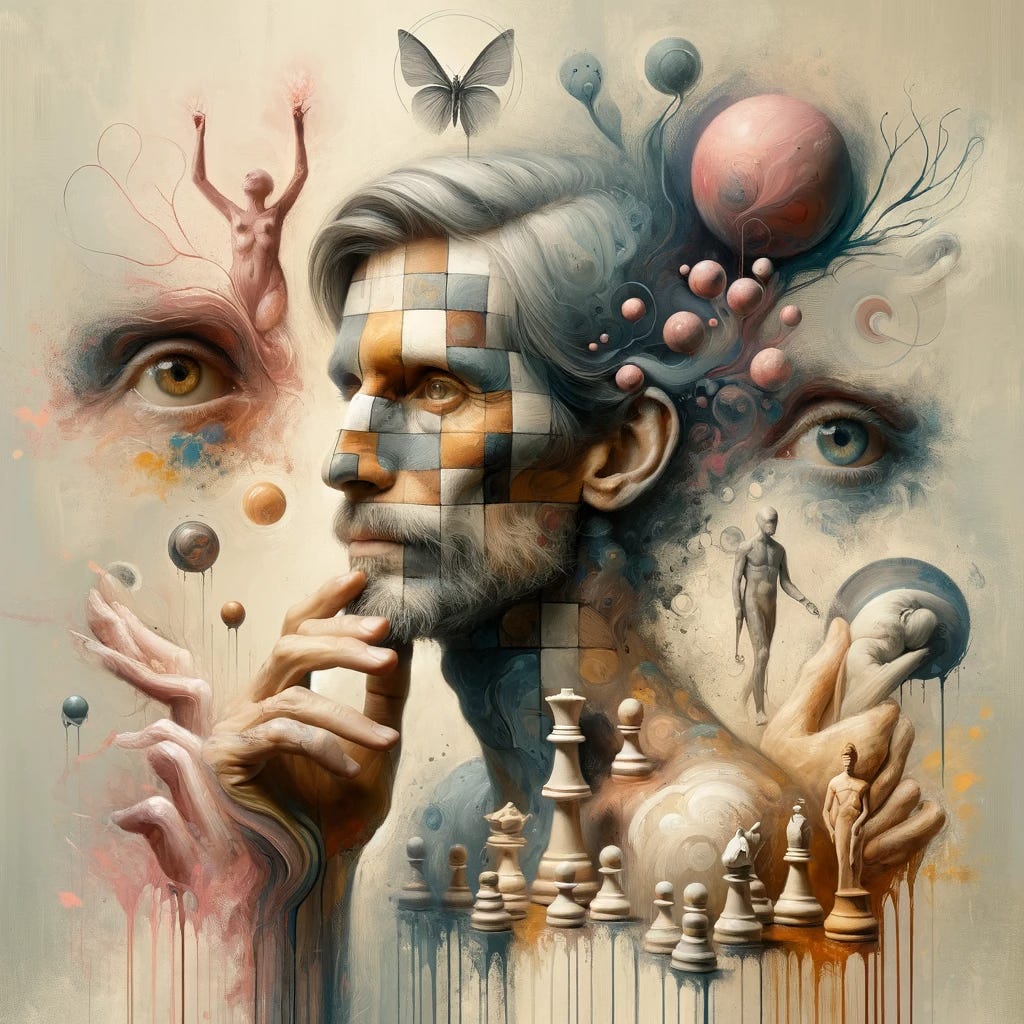This abstract artwork features a side profile of a contemplative man with silvery gray hair and a light-colored beard, set against an off-white taupe cream background. His face and neck are adorned with a multi-colored checkerboard pattern, featuring squares in blue, white, tan, gray, orange, and occasionally dripping with paint. The man's hand is raised to his chin in thought, and he gazes to the left. Below his shoulder, several chess pieces are clustered, adding a sense of strategic depth to the piece. Scattered throughout and surrounding the man are various disjointed elements: an image of a butterfly above his head, a realistic eye on either side of the composition—one blue on the right, one light brown on the left—and multiple human-like figures. Among these figures, a nude female, hands raised and gazing skyward, stands to the left. There are also fragmented hands and smaller round objects that resemble balls or beets interspersed throughout. Adding to the complexity, the artwork features sporadic watercolor splotches, enhancing its layered and textured appearance.